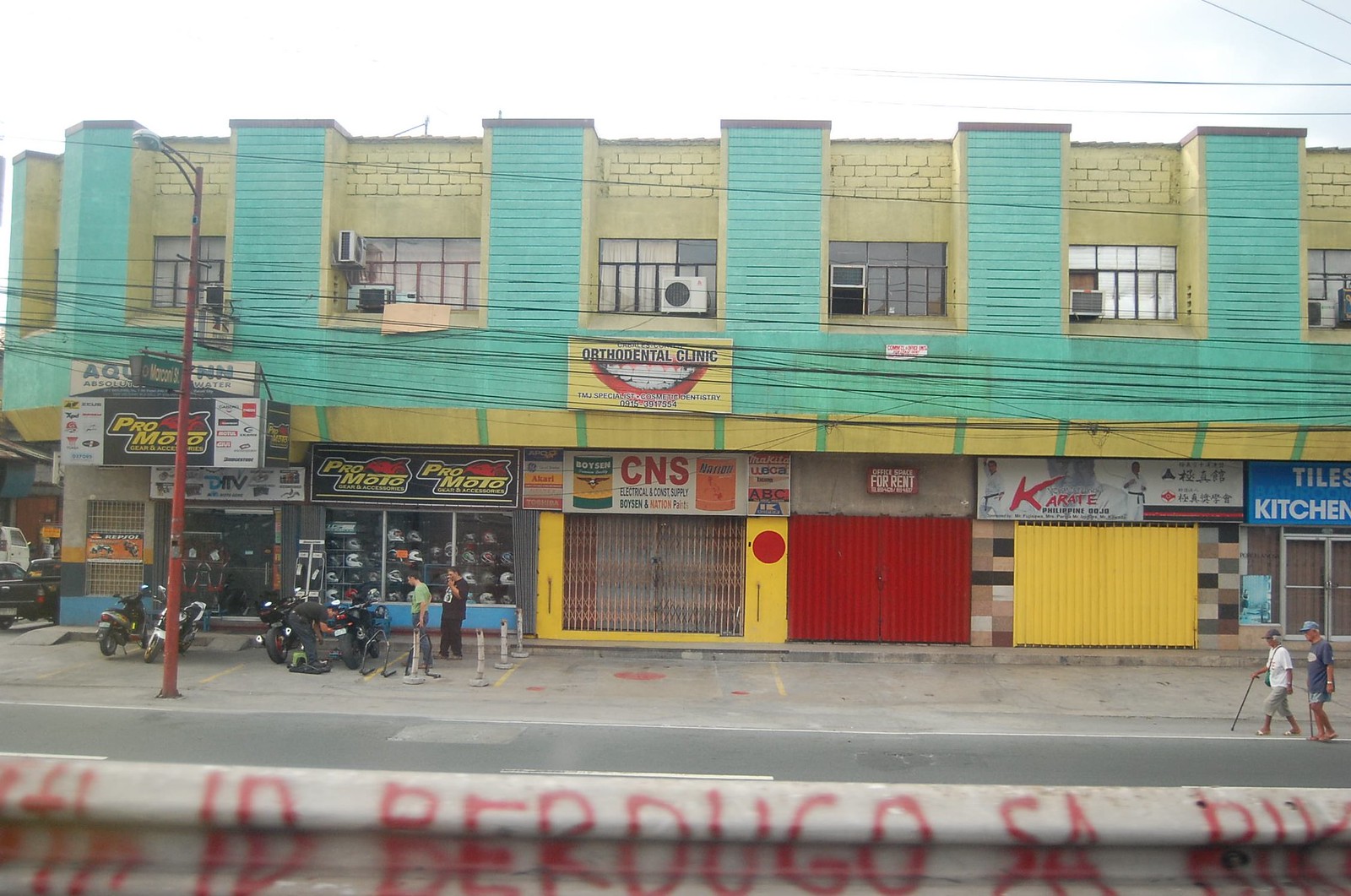The photograph captures an outdoor scene in what appears to be a different country. The focal point is a large, interconnected cement building situated along a gray roadway. The weather seems overcast or gloomy. The top portion of the building is painted in a combination of yellow and a unique shade of teal green. Each window on the upper levels has an air conditioning unit, suggesting they might be apartments.

The bottom section of the building houses various storefronts. Notable among these is a motorcycle store named Pro Moto, identifiable by helmets displayed in its window. Next to it is a boarded-up shop that once sold electrical supplies, labeled CNS Electrical and Cost Supply. There's also a karate studio and a tile and kitchen store. A centrally displayed poster advertises an orthodontic clinic, and a "For Rent" sign is visibly posted in one of the windows.

In the scene, people are walking along the road, some standing near the shops, while others cross the street. There are two-wheelers parked on the left side, alongside a tall lamp post. Electric cables stretch from left to right across the image, and some graffiti is visible on the building's surface. A few other illegible texts are painted at the bottom of the image, hinting at a certain local flavor in the setting.